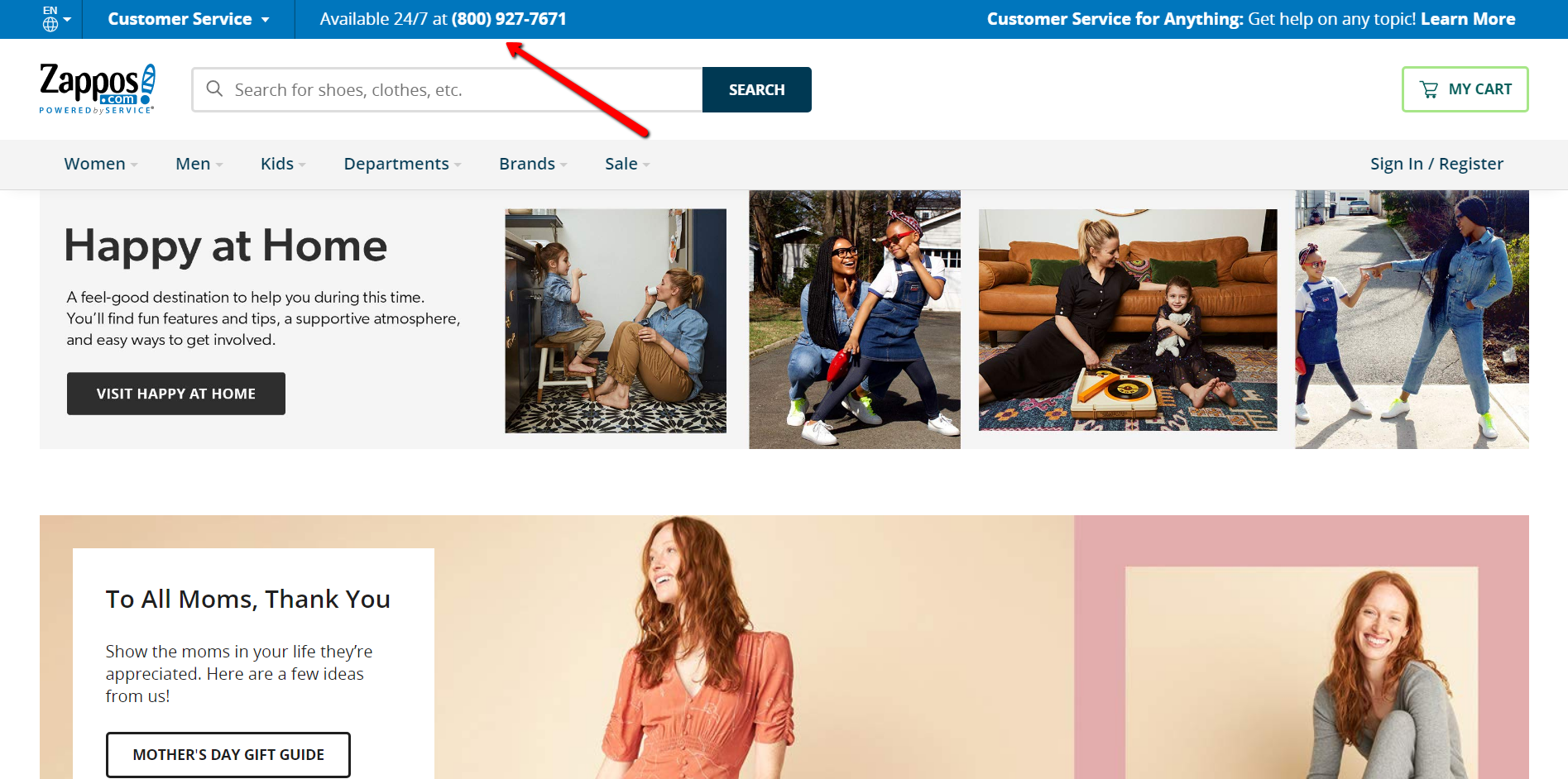The homepage of the Zappos.com website features a prominently displayed logo on the top left corner. This logo creatively incorporates an exclamation point that resembles the sole of a shoe with a curved area containing a "Z". Below the logo, the tagline "Powered by Service" is displayed. 

At the top of the page is a blue navigation bar with various options. On the left side, it includes a language selector displaying "EN" with a globe icon and a pull-down menu. Adjacent to this, there is a customer service section available 24/7, highlighted with a red arrow pointing to the contact number 800-927-7671 for assistance on any topic.

Next to the customer service information, a search bar is placed prominently with a blue button to initiate the search. On the far right side, there is a "My Cart" icon outlined in green.

Below the top navigation bar, various navigation tools are available including categories like "Women", "Men", "Kids", "Departments", "Brands", and "Sale", each accompanied by a pull-down menu for easy access.

A special section titled "Happy at Home" is advertised as a feel-good destination aimed to support and offer tips during challenging times. This section encourages visitors to explore content designed to enhance their well-being. Beneath this, there is a black button labeled "Visit Happy at Home".

An image of a mother and her daughter enjoying a tea party on the kitchen floor is featured, both dressed in matching outfits, adding a warm and welcoming visual element to the website.